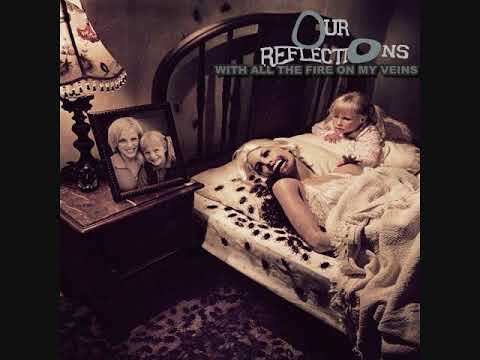The image, appearing almost black and white with dark, muted colors, portrays a disturbing bedroom scene. A woman with loose blonde hair and wearing a white nightgown lies in bed, partially covered by white sheets. Her face, tilted towards the camera, is marred by an unnatural, skeletal appearance, with her lips seemingly eroded away, leaving her mouth grotesquely open. Out of her mouth and crawling over her body and the bed are numerous bugs, including cockroaches and possibly leeches or spiders. Beside her on the bed, a little blonde girl with her hair in a ponytail, dressed in long sleeve pajamas or a nightgown, seems to be reaching out or observing her mother with a distressed expression, suggesting she is checking if her mother is alive. Above them, the words "our reflections with all the fire in my veins" are inscribed. On the left side of the bed, a wooden nightstand holds a Victorian-style lamp with bead-fringed edges and a framed photograph of the woman and child in happier times. The haunting and eerie scene is further intensified by the bugs creeping up the walls.